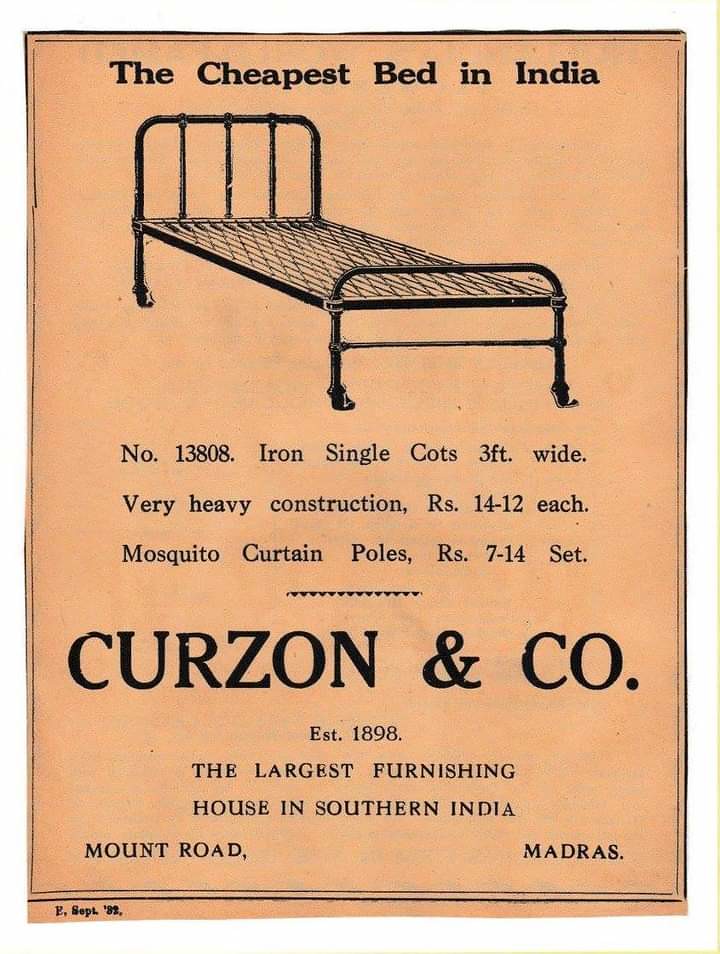This vintage advertisement is presented as a drawing on an orange background with prominent black lettering. It promotes Curzon and Company, established in 1898, which is described as the largest furnishing house in Southern India. The text boldly announces the product: "The cheapest bed in India," specifically item number 13808, an iron single cot that is 3 feet wide with very heavy construction, priced between RS 12 to 14 each. It also mentions mosquito curtain poles available in sets, priced from RS 7 to 14. The cot, shown in a black illustration, features the headboard, footboard, and frame, but no mattress. Additional text includes the company's address on Mount Road, Madras. In the bottom left corner, there is text that reads "E September 33." The overall layout suggests a straightforward and utilitarian advertisement, probably designed for a newspaper or poster.